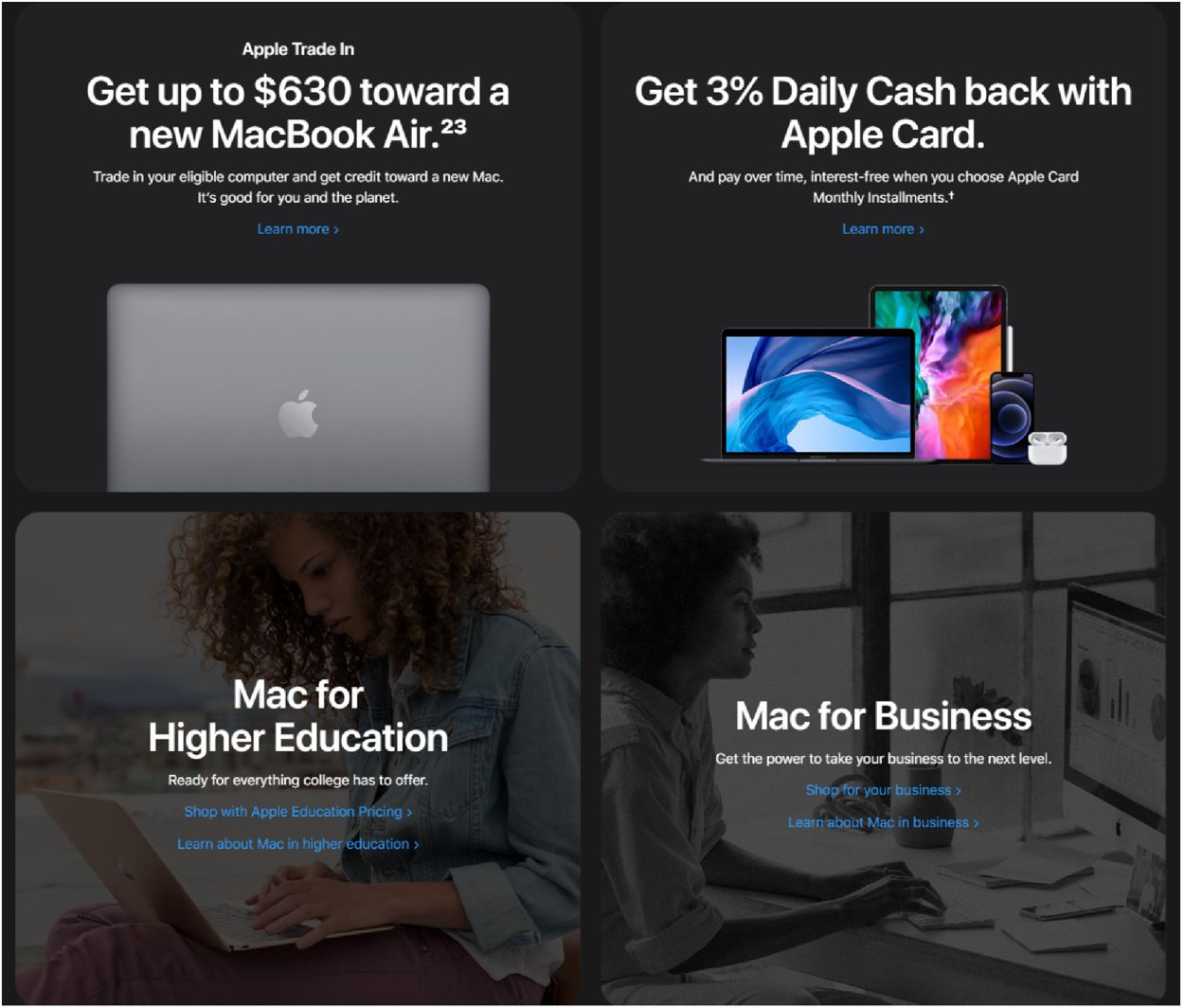This screenshot features a black background divided into four quadrants, each with varying details and imagery. 

**Top Left Quadrant:**
- The text "Apple Trade-In" is centrally displayed in white.
- Below it in larger white text: "Get up to $630 toward a new MacBook Air."
- A small "23" appears at the end of this line.
- Further below in smaller white text: "Trade in your electric computer and get credit towards a new Mac."
- This is followed by: "It's good for you and the planet."
- Centered in blue text is: "Learn more" with a right arrow.
- Below that is a gray rectangle, representing the back of a laptop screen with an Apple logo centered.

**Top Right Quadrant:**
- The text "Get 3% daily cash back with" is centered in white.
- Below that: "Apple Card."
- In smaller white text: "And pay over time, interest-free when you choose Apple Card monthly installments."
- Centered in blue text: "Learn more."
- Below this text is an image of a laptop screen, a tablet screen, and a cell phone, each displaying colorful screensavers.

**Bottom Left Quadrant:**
- Shows an image of a woman with a laptop on her lap in the background.
- Centered, bold text: "Mac for Higher Education."
- Below in white: "Ready for everything college has to offer."
- Two lines of blue print appear below this.

**Bottom Right Quadrant:**
- Features a picture of a woman sitting at a desk working on a desktop computer.
- Centered white text: "Mac for Business."
- Below: "Get the power to take your business to the next level."

Each quadrant effectively highlights various promotional aspects and product details available through Apple, addressing trade-ins, financing options, educational benefits, and business applications.